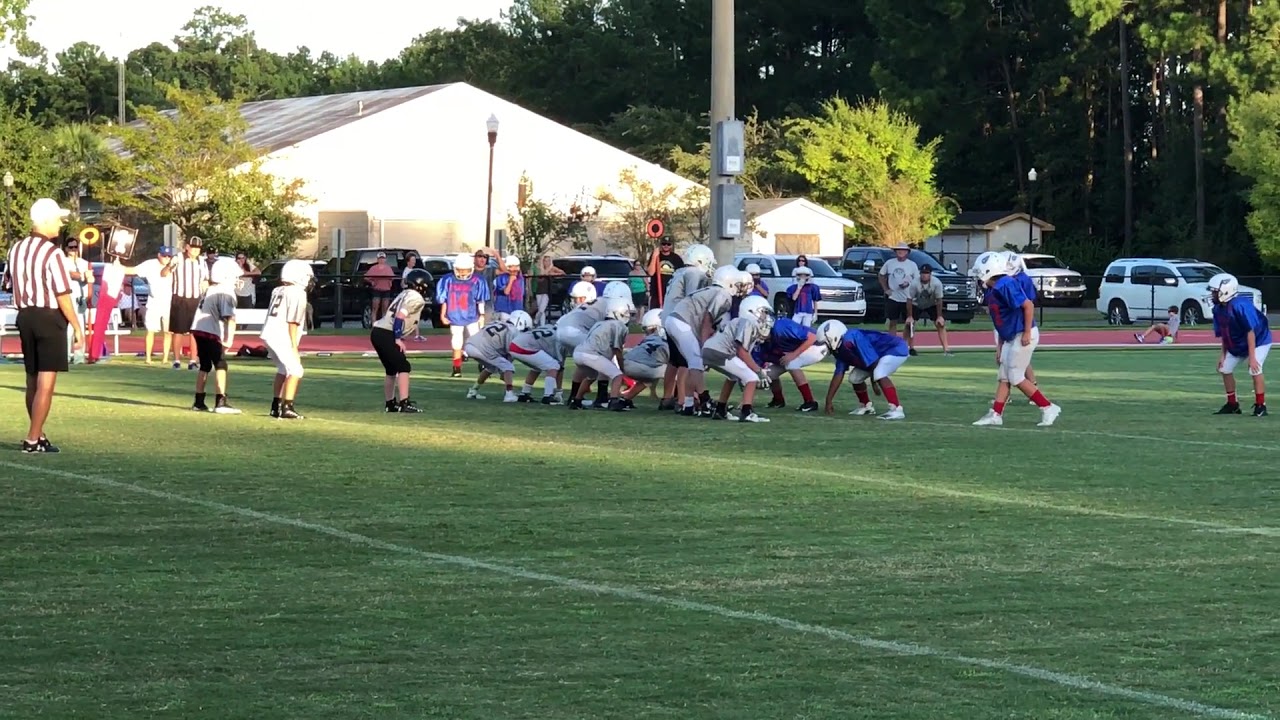The image depicts an outdoor football game on a large green field, likely at a school, as evidenced by the surrounding red clay-colored running track. The teams are facing each other in the ready position for a play, with the offensive team on the left dressed in all white uniforms and helmets. The defensive team, on the right, wears blue jerseys with white pants and helmets featuring a blue logo. Two referees are visible; one on the far left of the picture and another further back. There are vehicles parked in a nearby lot and a white building, possibly residential, is seen in the background along with numerous tall green trees. A pole, possibly for overhead lights, stands just behind the players, further enhancing the scene's outdoor and spacious setting.